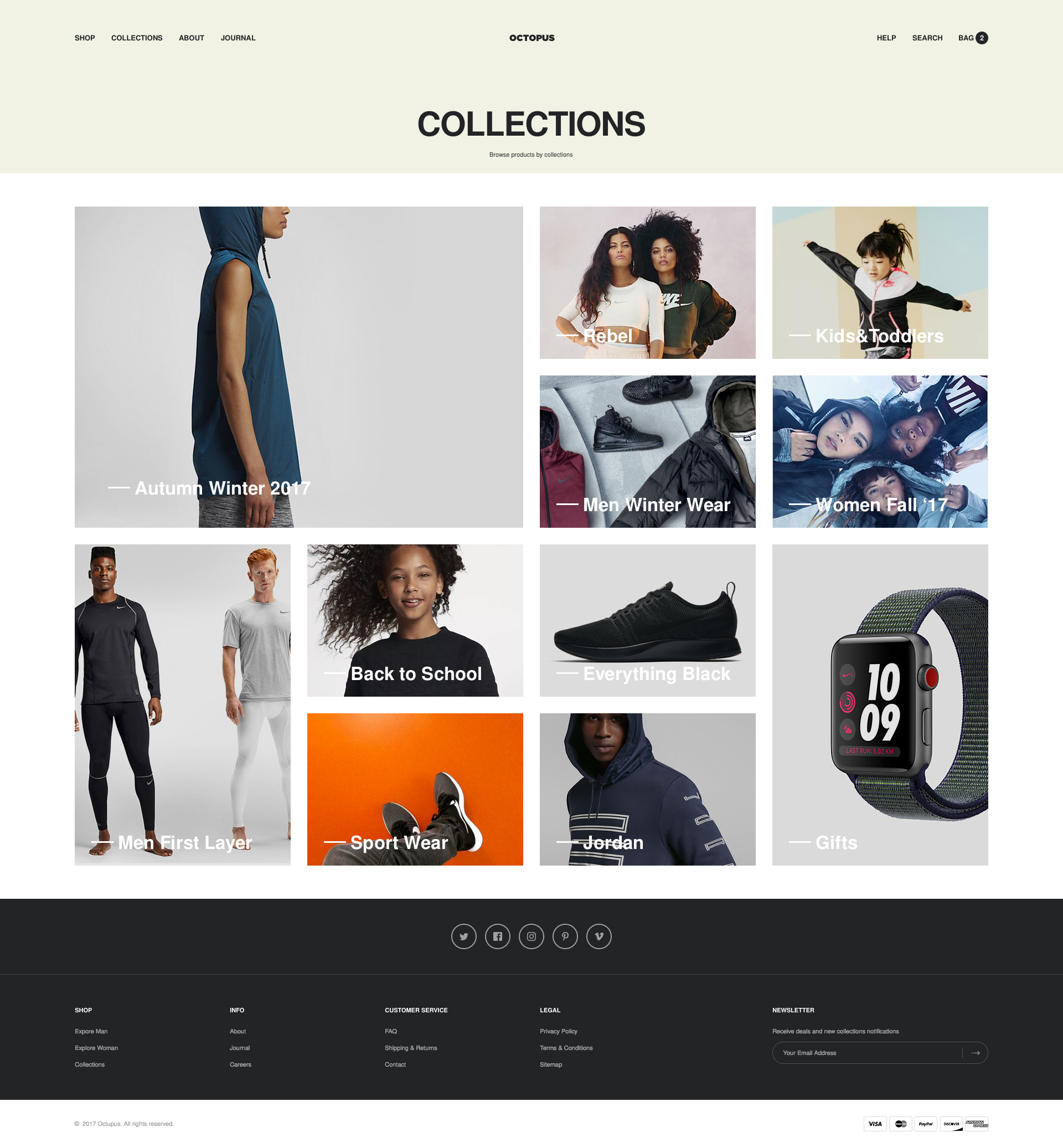Explore the meticulously curated shopping website for the store called Octopus. The header gracefully rests against a light beige background, featuring the store's name, "Octopus," in small black letters. The navigation bar provides seamless access to shop collections, an about journal, help options, a search bar, and your shopping bag.

Beneath the header, the word "Collections" is prominently displayed in larger, black, capital letters, guiding your gaze to an array of inviting images showcasing the diverse products on offer. Embark on a visual journey through their categories: 

- **Autumn/Winter 2017:** A cut-off image of a man donning a cozy hoodie.
- **Rebel, Kids and Toddlers:** A lively selection for the young ones.
- **Men’s Winter Wear:** Warm and stylish apparel for men.
- **Women’s Fall 2017:** Trendy and chic autumn attire for women.
- **Everything Black:** Featuring a sleek black shoe.
- **Back to School:** A vibrant image of a teenager, capturing the spirit of the season.
- **Men’s First Layer:** Showcasing a practical black insulated shirt, ideal for layering in winter.
- **Sportswear, Jordan:** Athletic wear for active lifestyles.
- **Gifts:** A thoughtful selection epitomized by an image of a smartwatch.

At the page's end, a sleek black box offers additional options, inviting users to sign up for the newsletter, follow Octopus on social media, or explore various legal options.